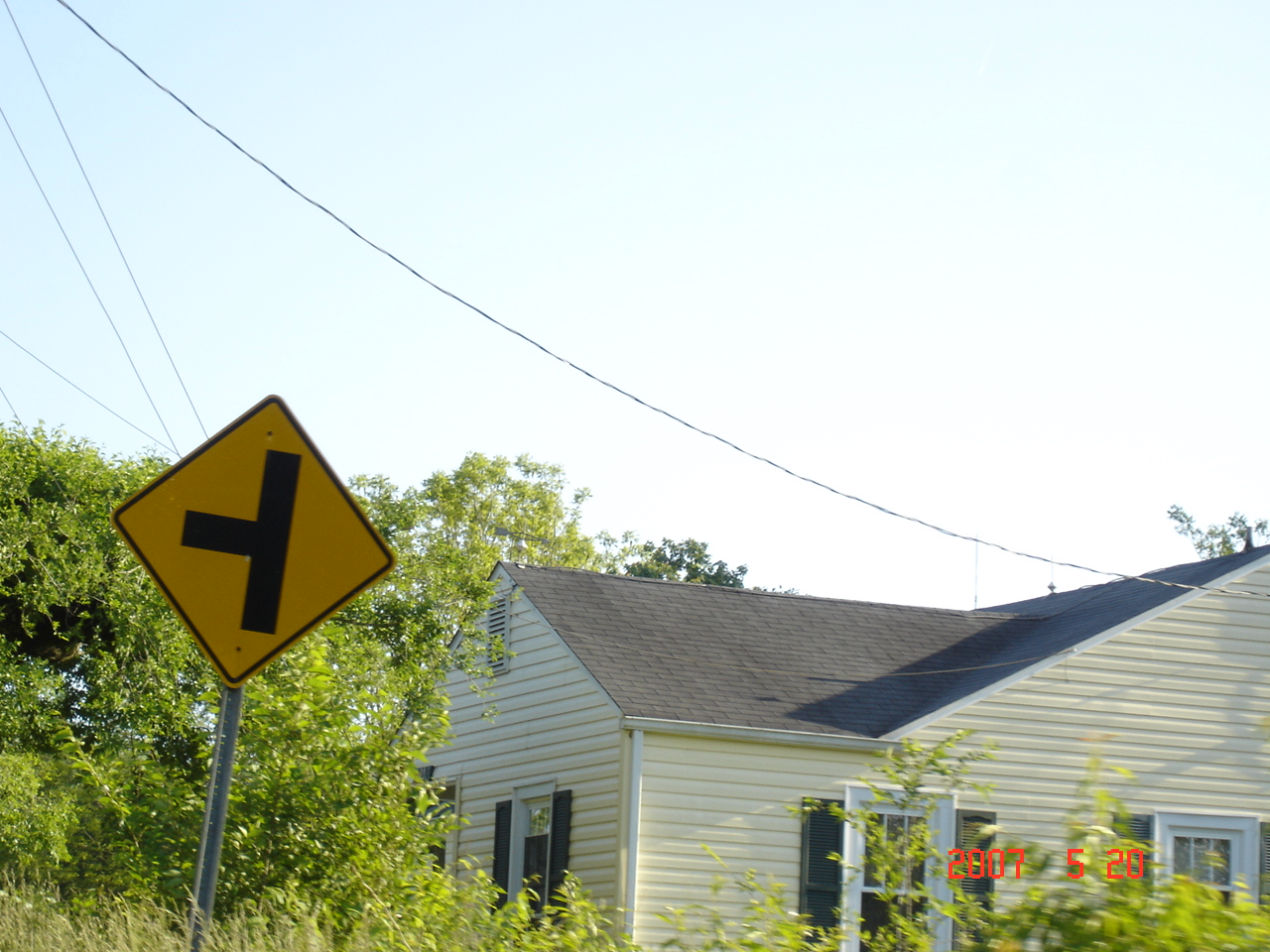A photograph captured from the sidewalk shows the exterior of a home on May 20th, 2007, as indicated by an orange timestamp in the bottom right corner. The house is adorned with either white siding or a very pale yellow or cream-colored siding. It features white painted window frames paired with black shutters. The architectural style of the house is unclear, leaving it ambiguous whether it is a one-story or a two-story structure. 

Surrounding the house are numerous trees, providing a lush backdrop, while the front yard is landscaped with various green plants and shrubs. A gray metal pole stands adjacent to the home, bearing a yellow diamond-shaped street sign that signifies a T intersection with a bold black vertical line and a connecting line to the left. The pale blue sky casts a shadow across the facade, with multiple telephone wires crisscrossing above the house, adding to the suburban setting.